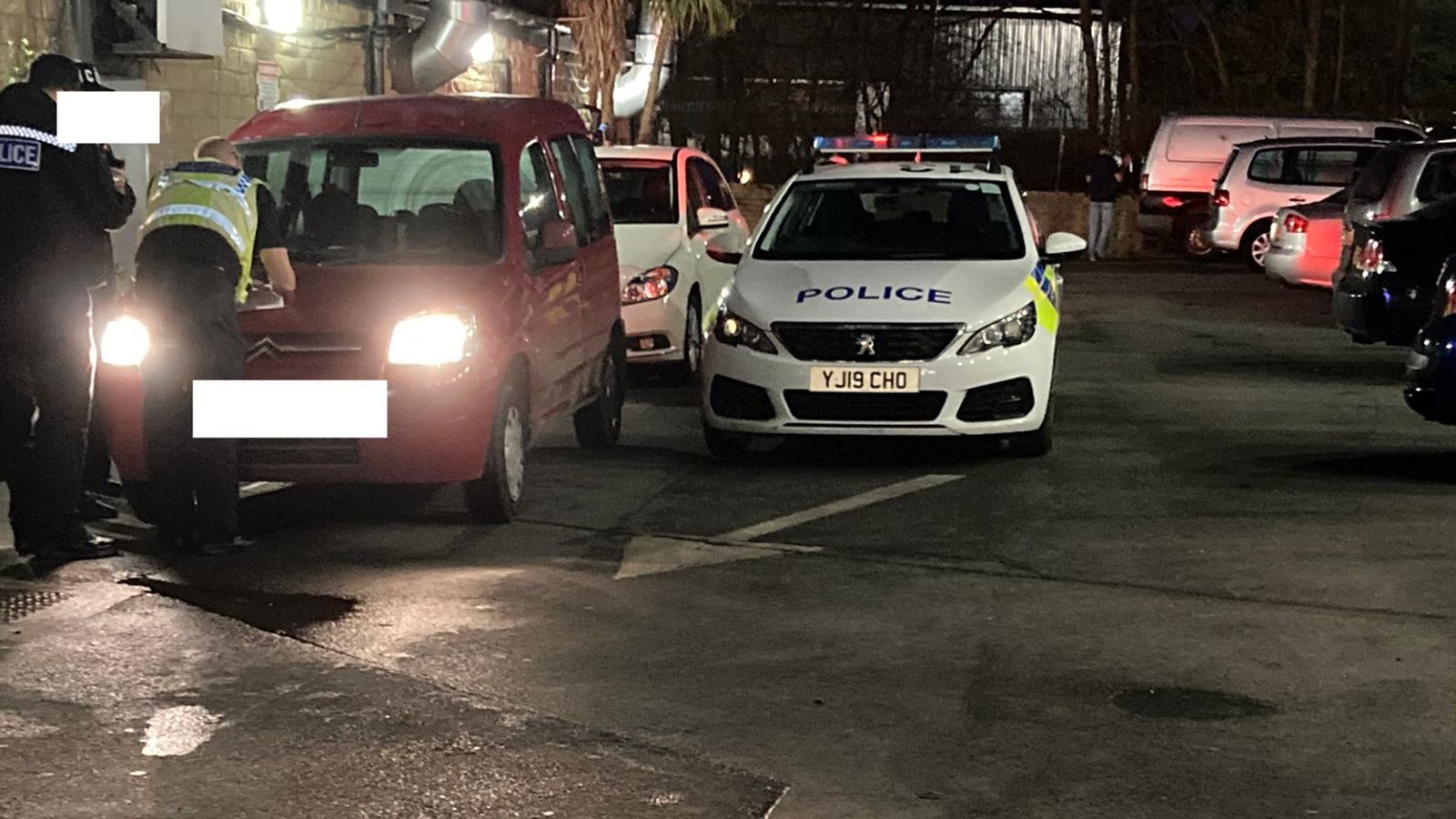This nighttime photograph, set in a wet parking lot evident by the glistening asphalt, captures a European police encounter. Dominating the scene is a white police car with dark lettering on the front, and a license plate indicative of Europe. Surrounding the police vehicle are six other cars, highlighted by a red compact car on the left side of the image with its headlights on. Leaning over the hood of this red car, which was likely pulled over, is a police officer in a reflective yellow and white vest, busy writing something down. Adjacent to him stands another officer in a black uniform with white stripes, his face obscured. The background fades into darkness, with faint reflections hinting at more distant activity. Across from the police car, arranged in perpendicular parking, are four more vehicles. An arrow on the pavement directs traffic flow, while subtle red lights in the background hint at other vehicles. The scene’s focus is squarely on the police interaction, underscoring the seriousness of the moment amidst the quiet night setting.